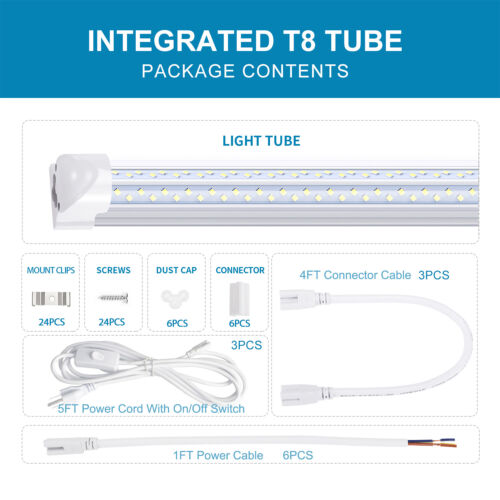The image showcases an advertisement for an integrated T8 light tube set against a white background. At the top, a blue banner with bold, all-caps white text prominently reads "INTEGRATED T8 TUBE." Beneath this, in a regular blue font, the text states "Package Contents."

Centered below is a grey-dotted bordered image. In blue capital letters, it reads "Light Tube," illustrating a horizontal light tube with yellow triangular designs representing the lights, accompanied by a white component on the left.

Further down, a detailed list and corresponding images display the package contents, all in blue font:
- 24 Mount Clips
- 24 Screws
- 6 Dust Caps
- 6 Connectors
- 3 Four-Foot Connector Cables
- 3 Five-Foot Power Cords with On/Off Switch

At the bottom, a horizontal image spans the entire width, showcasing a "1 Foot Power Cable, 6 inches" label. The depiction features a white cable running horizontally from left to right, with a black wire extending from it, marked by a small yellow segment, and a red wire with a thinner red portion.

This comprehensive visual ensures clarity on the included components, aiding consumers in understanding the package contents effectively.